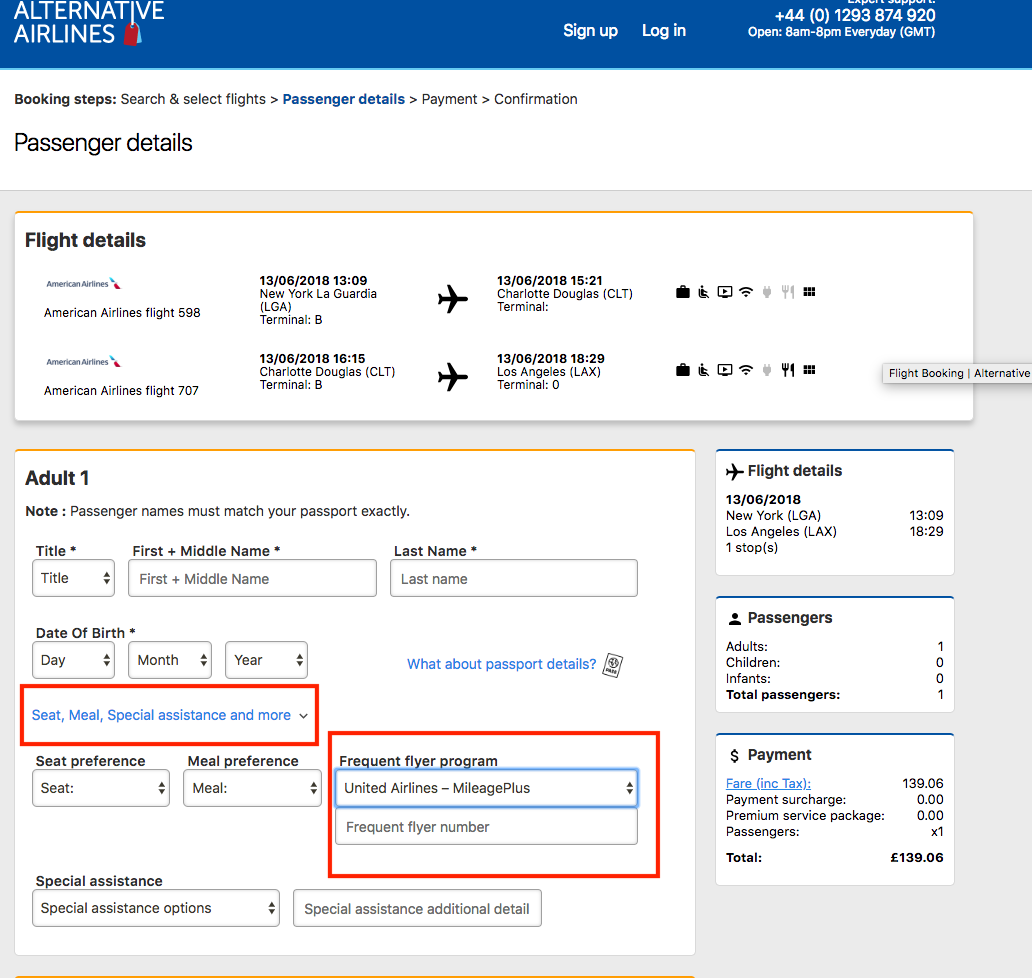This screenshot displays a detailed section of the Alternative Airlines website. At the top, a blue navigation bar features the company's name, "Alternative Airlines" in white font on the upper left corner, alongside an icon of two luggage tags—one red and one white—dangling from the letter "I" in "Alternative." Centrally positioned on this blue bar are links for "Sign Up" and "Log In". On the far right, it lists contact information as "+44 (0) 1293 874 920" followed by the operating hours, "Open: 8 a.m. to 8 p.m. every day, GMT".

Below the blue navigation bar is a white bar displaying the booking progression steps in black font: "Booking Steps" followed by "Search and Select Flights," and an arrow pointing to "Passenger Details," which is highlighted in blue. Subsequent steps listed are "Payment" and "Confirmation," each separated by a forward arrow, indicating the user is currently on the "Passenger Details" page.

The main content area, which is gray, contains a white rectangular section at the top labeled "Flight Details." Here, two American Airlines flights are listed: Flight 598 from New York LaGuardia and Flight 707 to Charlotte Douglas.